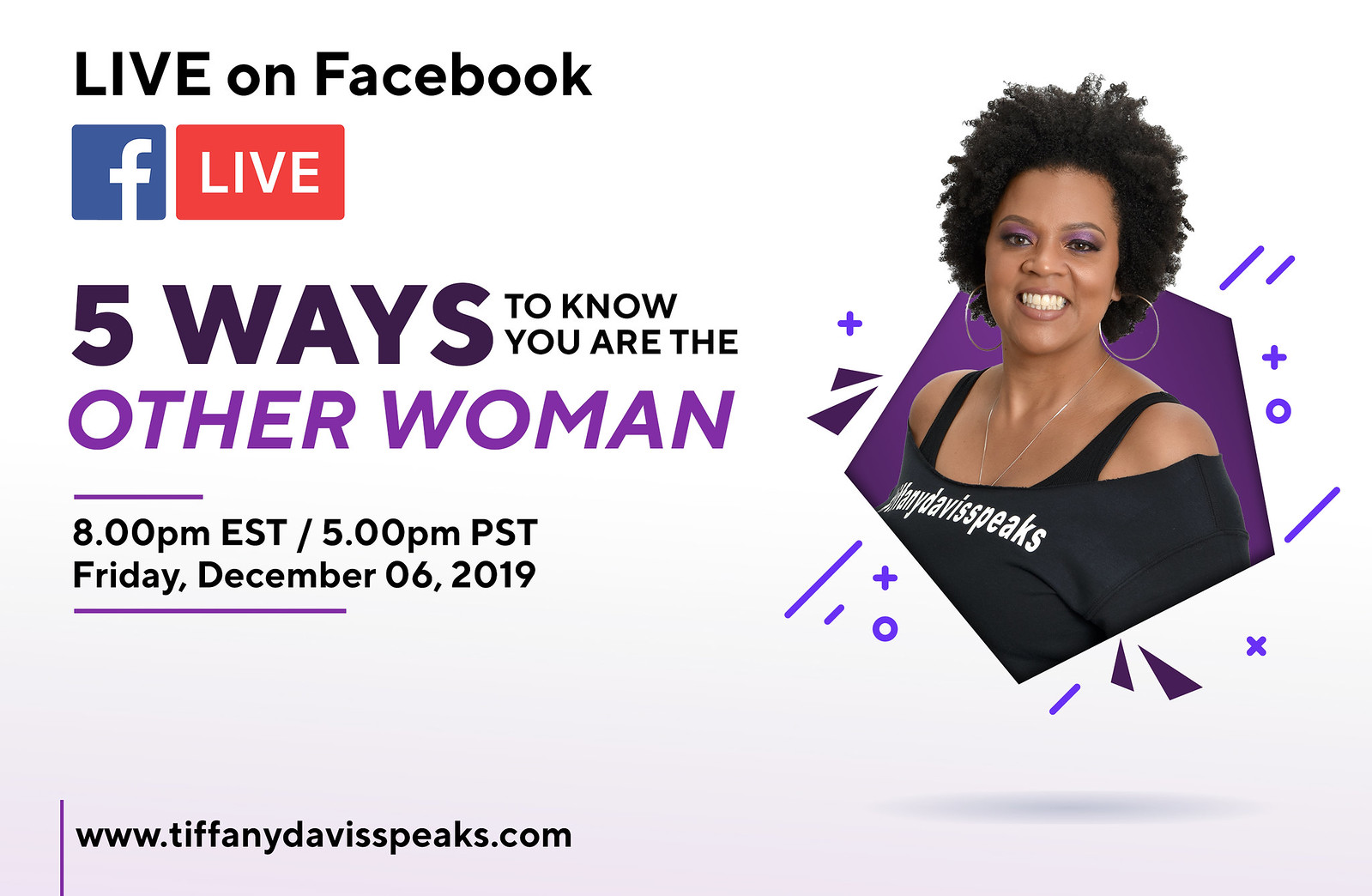The poster features a sleek, all-white background with a clear advertisement for an upcoming live event on Facebook. In the upper left-hand corner, it states "Live on Facebook" in black lettering, accompanied by the blue-and-white Facebook logo and a red "Live" icon. Directly beneath this, the event title "Five Ways to Know You Are the Other Woman" is prominently displayed, with "the other woman" highlighted in a brighter purple against a dark purple background. The event details are provided below in black text: "8 p.m. Eastern Time, 5 p.m. Pacific, Friday, December 6, 2019."

To the right of these details is a photograph of the speaker, Tiffany Davis, a black woman with short dreadlocks. She is wearing large round hoop earrings, a black tank top, and a black off-the-shoulder blouse featuring the words "Tiffany Davis Speaks." Her image is set against a purple geometric shape, either a triangle or hexagon. In the lower left-hand corner, the website "www.tiffanydavisspeaks.com" is clearly listed.